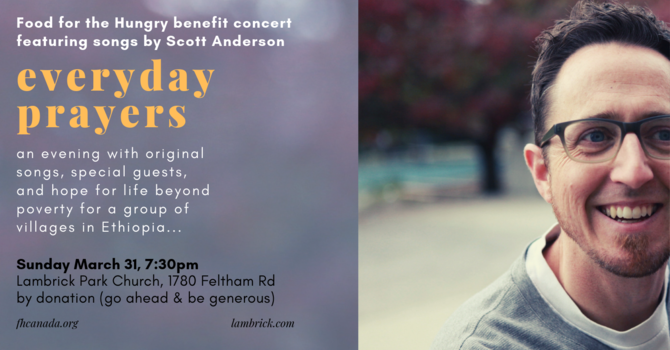This image is an advertisement for a church event called "Everyday Prayers," a benefit concert organized to support "Food for the Hungry" and provide hope for life beyond poverty for a group of villages in Ethiopia. The left side of the image features a gray and purplish-blue background with white, yellow, and black text. At the top, in white text: "Food for the Hungry Benefit Concert featuring songs by Scott Anderson." Below that, in yellow text: "Everyday Prayers." Continuing in white text: "An evening with original songs, special guests, and hope for life beyond poverty for a group of villages in Ethiopia." Further down, in black text, the details of the event: "Sunday, March 31st, 7:30 p.m. Lambrick Park Church, 1780 Feltham Road. By donation, go ahead and be generous." Additionally, URLs for FHCANADA.org and lambrick.com are displayed. 

On the right side, there is a photograph of a smiling white man, presumably Scott Anderson. He appears to be in his 30s, has brown hair and black-rimmed glasses, and is wearing a gray sweatshirt over a white shirt. The background of the photograph is blurry but suggests an outdoor setting with a tree having red and green leaves.